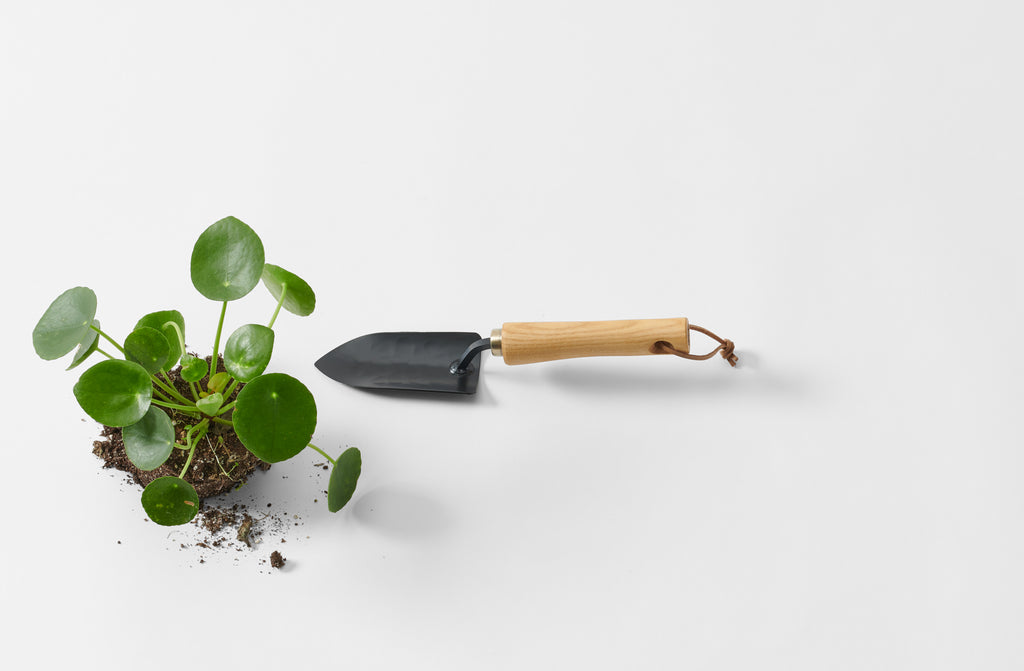A freshly dug-up plant with round leaves sits on a pristine white surface, its roots encased in a neat, spherical clump of soil. Beside it lies a small gardening hand spade, with a metal blade that is straight on the right side and tapers to a point on the left. The spade features a wooden handle, which has a hole at its end threaded with a piece of leather string, tied off to allow for convenient hanging. The hand spade is positioned to the right of the plant, adding a touch of rustic charm to the scene.